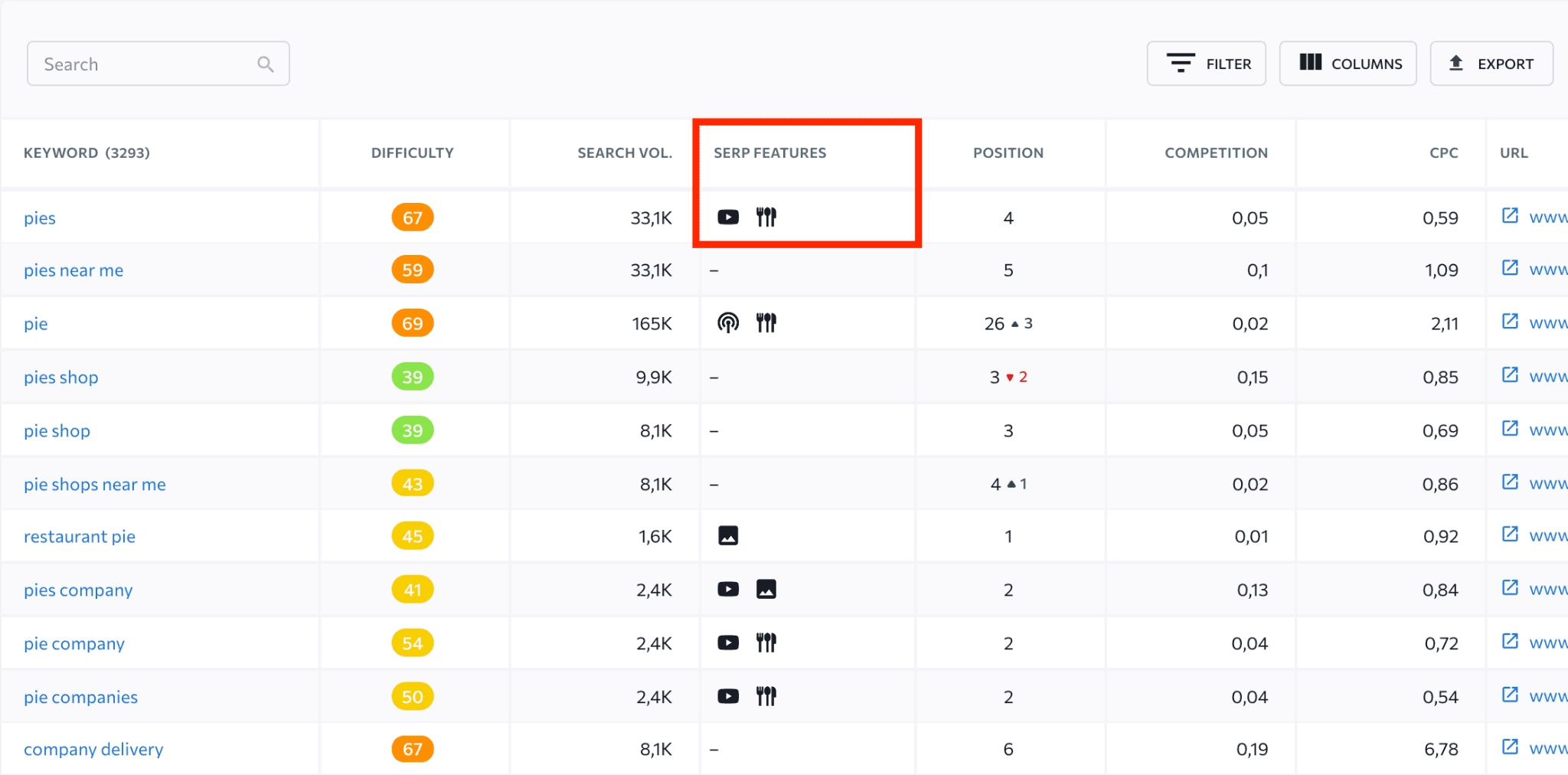A detailed caption for the image provided could be:

"An image of a detailed search engine optimization (SEO) spreadsheet is displayed, primarily featuring black text on a white background. The top left corner contains a search box, while the top right corner includes options for filtering, selecting columns, and exporting data. The spreadsheet consists of multiple columns, each with specific information.

The 'Keywords' column lists various search terms, including 'pies,' 'pies near me,' 'pie shops,' and 'restaurant pie.' Adjacent to these keywords, there are rounded squares in the 'Difficulty' column, showcasing numeric values with color-coded backgrounds: orange (67, 59, 69), green (39, 39), yellow (43, 45, 41, 54, 50), and orangey-red (67). 

In the 'Search Volume' column, figures range from approximately 33,000 searches at the top to about 1,600 at the bottom. The 'SERP Features' column is highlighted with a red border and includes various icons such as a Google Play symbol, cutlery, Wi-Fi/mobile hotspots, images, and play buttons.

The 'Positions' column reflects the ranking of each keyword, with numbers such as 64, 5, 26, 3, 3, 2, 3, 4, 1, 1, 2, 2, 2, and 6. The 'Competition' column indicates very low values, starting at 0.05 and slightly increasing to 0.1. The 'CPC' (Cost Per Click) column starts at 0.59 with its highest value at 6.78 at the bottom.

On the far right, a list of web addresses is partially visible, recognizable by the repeated 'WWW' prefix in blue text, although the full URLs are not entirely readable due to the image cut-off."